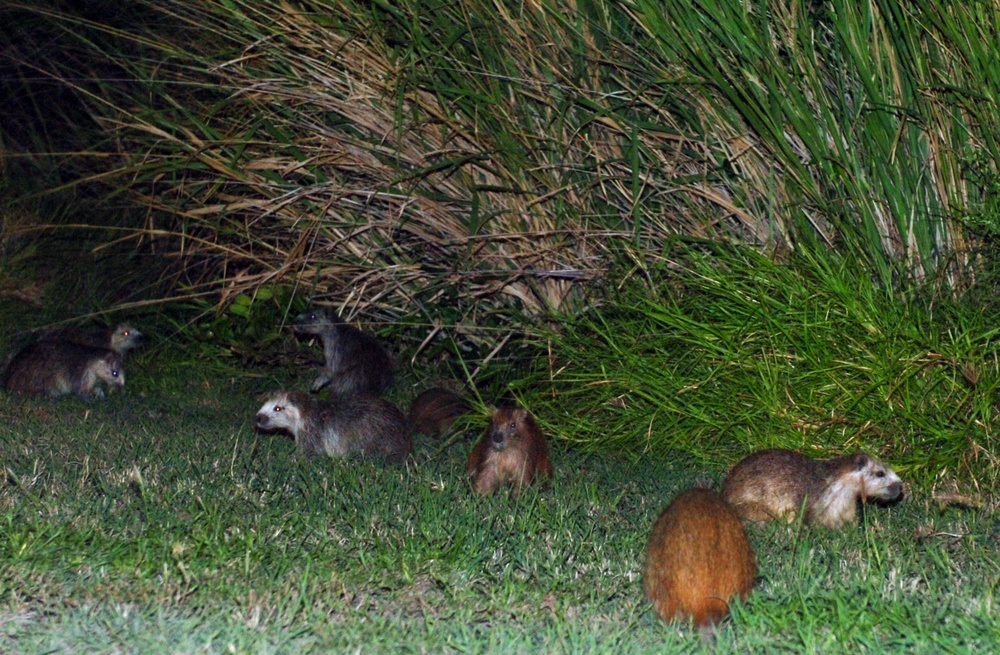This nighttime photograph captures a fascinating gathering of seven porcupines standing in a grassy area. The scene is set against a backdrop of tall, wild grasses that rise from the center of the image and stretch beyond the frame, with some of the foliage browning amidst the greenery. These porcupines, exhibiting a mix of gray and brown fur, are spread across the scene from left to right and are engaged in various activities. The group includes individuals with distinctive white fur on their faces, one with a fully brown coat observed from behind, and another with a blonde face. Their glowing eyes add an enchanting touch to the nocturnal ambiance. The porcupines are huddled closely, suggesting social behavior, under the imposing, wispy grasses.